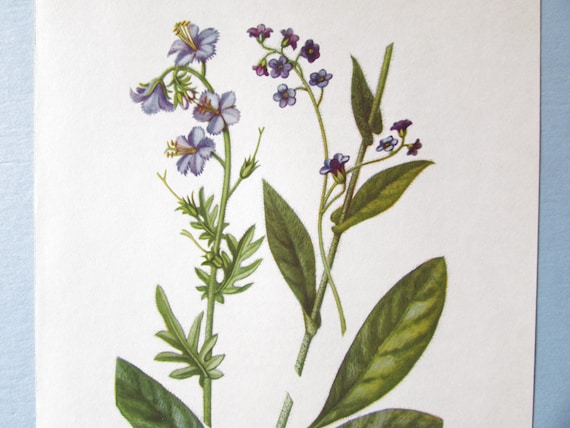This detailed artwork, either a painting or a hand drawing, showcases a complex and vibrant depiction of plant life, displayed on a thicker sketch paper against what appears to be a light blue, possibly plaster-like surface. The background of the artwork is white, bordered by darker blue margins on the left and the right sides. The drawing features a green stalk originating from the bottom left and rising to the top, adorned with various leaves and flowers. 

From the bottom of this stalk, a large green leaf extends leftward, followed by a smaller leaf with six lobes. Higher up, a similarly structured leaf juts out to the right. Above this are three twigs with unbloomed flower buds. Near the top, four purple flowers, each with about four to five petals and some hairy extensions, bloom from the sides, slightly spaced apart.

On the right side of the composition, another stem angles upwards, bearing leaves of varying sizes. Two large leaves extend from the bottom, with subsequent leaves of decreasing size positioned higher along the stem, all pointing upwards. Above these leaves, a secondary stem diverges, terminating in a cluster of six purple flowers. Midway, another smaller stem branches off to the right, adorned with four more purple flowers. This artwork captures the vibrancy and different stages of growth of the plant, with detailed and colorful leaves and flowers in various shades of green and purple.